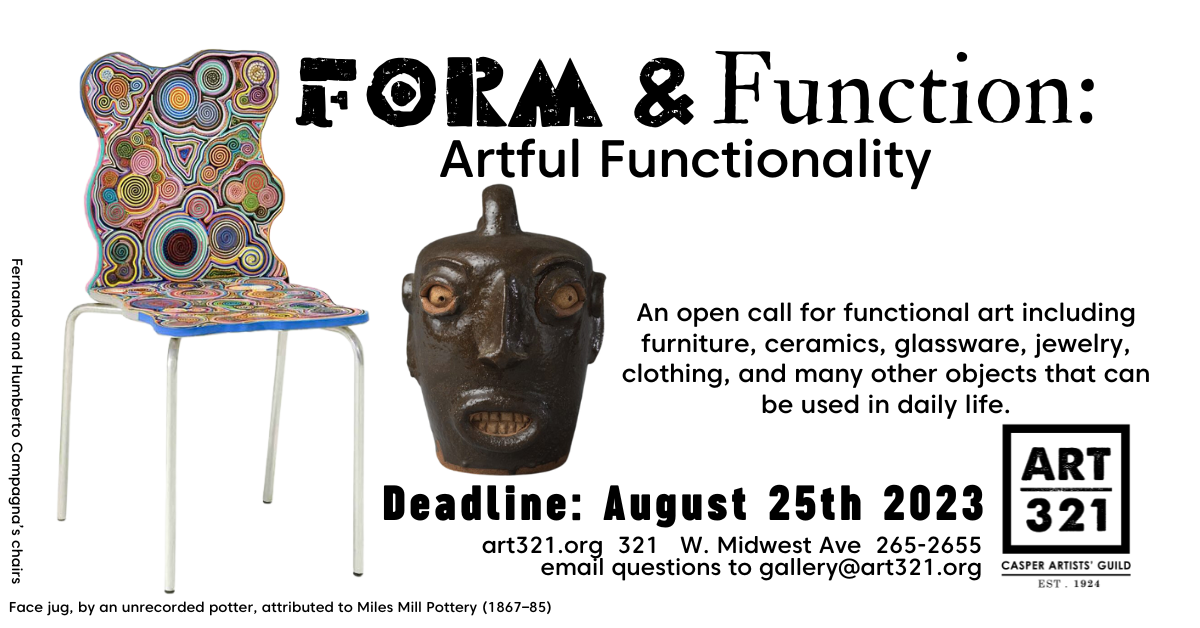An announcement flyer for a competition or display opportunity for artists sponsored by Art321, titled "Form and Function: Artful Functionality." The flyer invites artists to submit functional art pieces such as furniture, ceramics, glassware, jewelry, clothing, and various objects used in daily life. The deadline for submissions is August 25th, 2023. The event will be held at Art321, located at 321 Midwest Avenue in Casper. The flyer features a colorful, intricately designed chair with blue trim and thin silver legs, attributed to Fernando and Humberto Campana. Another illustrated item is a dark brown face jug resembling African tribal art with wide eyes and bared teeth, attributed to Miles Mill Pottery from 1867-85. The overall theme emphasizes the blend of form and function in artistic creations.